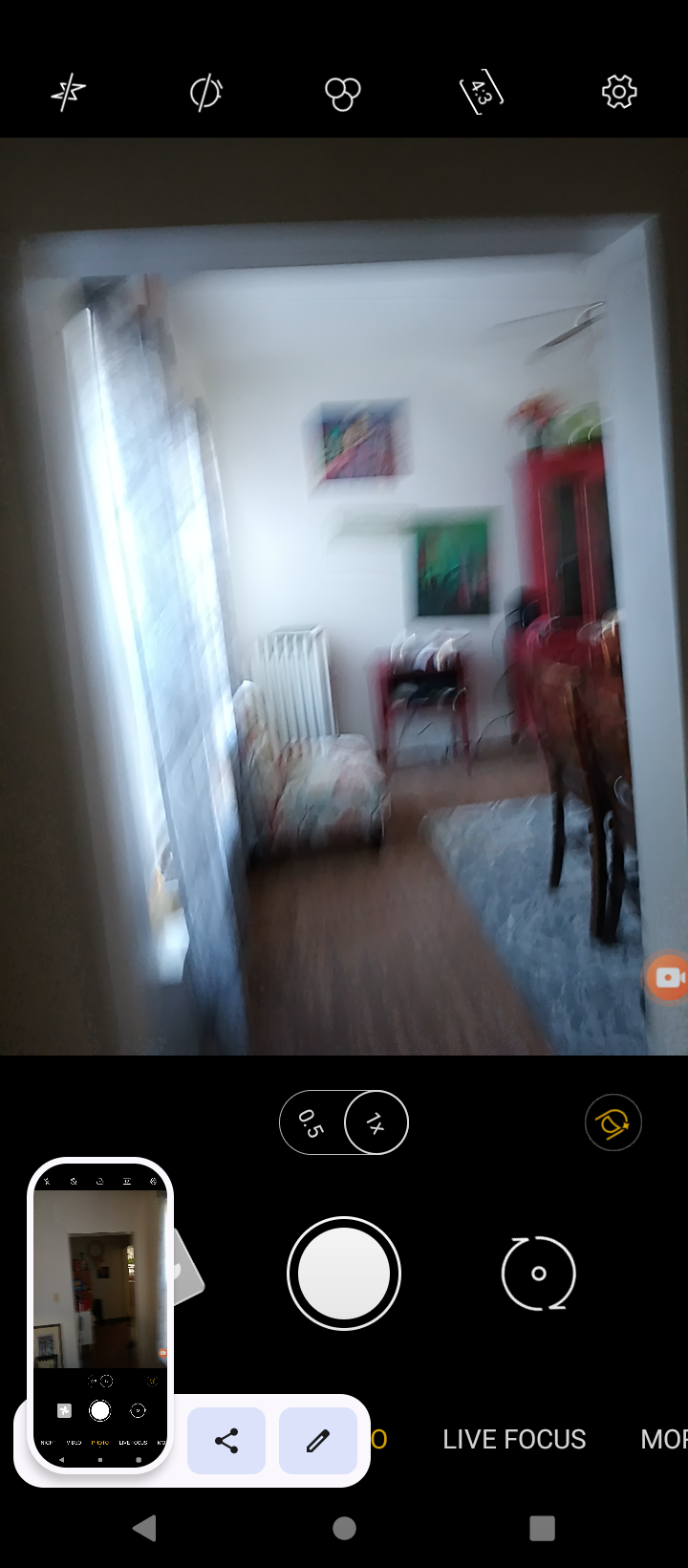This is a vertical, rectangular color photograph captured as a screenshot from a smartphone, possibly an Android device. The image prominently features the interface of a camera app, evident by the black borders at the top and bottom that contain various icons and settings, including the settings icon at the top right and a 'Live Focus' icon at the bottom. The central white circle at the bottom serves as the take picture button, flanked by other typical Android control icons such as the back button, home button, and recent apps button along with a play button in the center. 

The actual photograph depicted on the smartphone screen is a blurry image of a living room. The room has a hardwood floor of rich brown tones. On the right side of the image, part of a shaggy, sky-blue area rug is visible with the legs of a dark brown wooden chair resting on it. A darker red China cabinet with at least one potted flower, possibly dried, is situated against the left edge of the photo. Also notable on the left side is a white radiator that stands vertically up to about hip height. Light streams into the room from a window partially covered by long curtains, casting soft illumination across the floor. In the back corner, a light-colored wall is adorned with two posters, and just below them, a red object is discernible. Further in the background, near the white molding around an entryway, a low, cushioned chair without armrests is positioned.